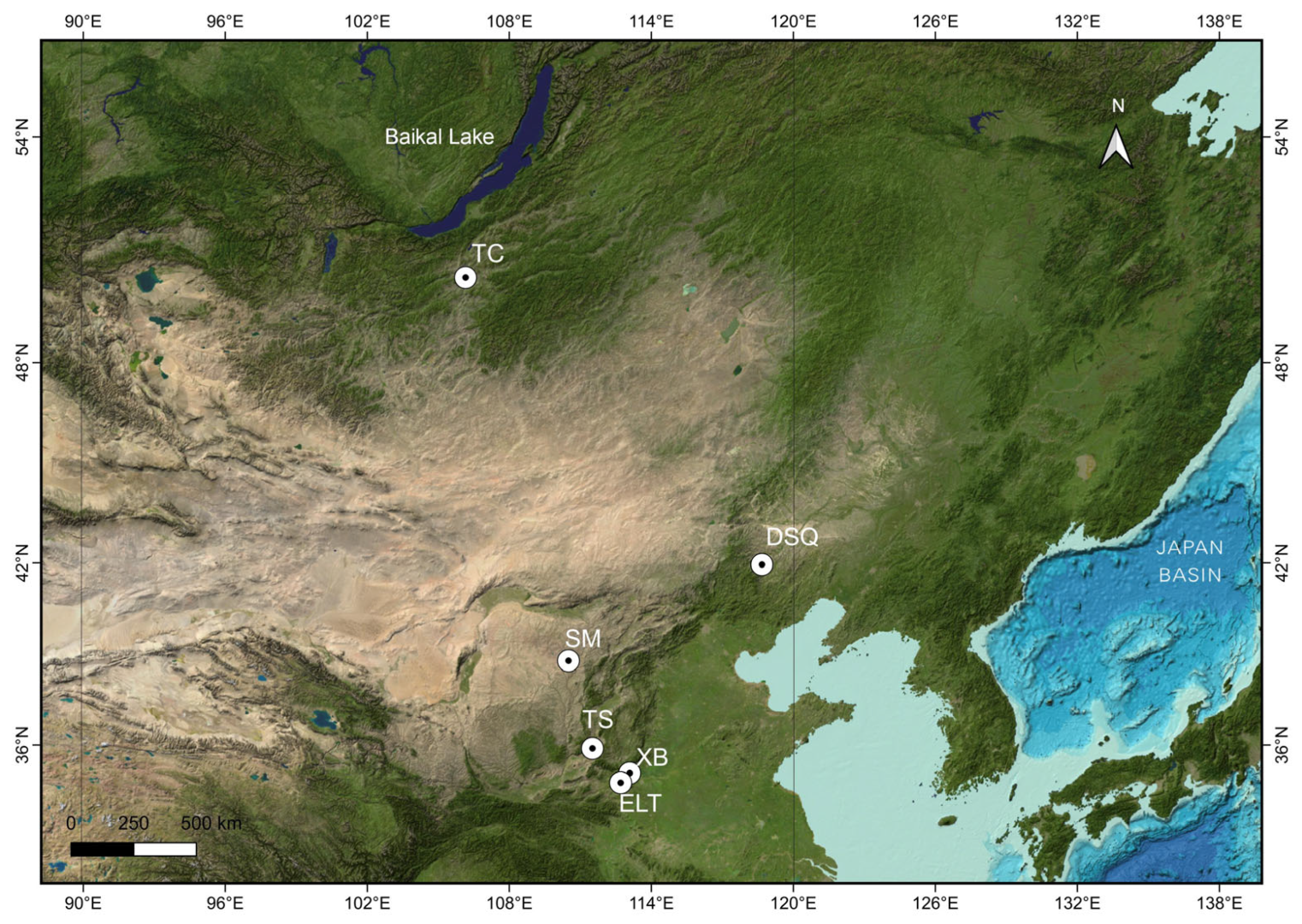This is a detailed aerial photograph of a landmass that appears to be part of the Asian continent. The map is bordered by longitude and latitude degrees: starting from 90 degrees east and incrementing by six to 138 degrees east along the top, and from 54 degrees north descending to 36 degrees north along the sides. A compass in the upper right corner indicates that north is at the top of the image. The bottom left corner contains a scale bar showing distances from 0 to 500 kilometers. 

Prominent features include Baikal Lake in the upper middle section, identified by a label, and the Japan Basin on the right, indicating a distinct body of water. Various points on the map are marked with abbreviations: TC south of Baikal Lake, ELT in the southernmost part, XB slightly northwest of ELT, TS northeast of XB, SM north of TS, and DSQ northeast of SM.

The land is predominantly green, suggesting lush vegetation, with some brown areas that may indicate mountains or deserts. The Japan Basin is noticeably blue, more so than other bodies of water, and the coastal areas are vividly green without brown edges.